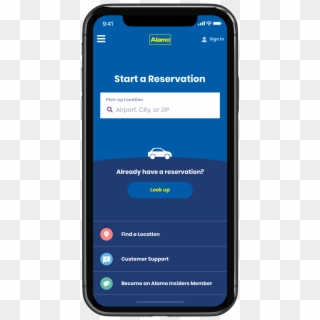This image is a digital mock-up of a smartphone screen designed for advertising Alamo car rentals. The background features a minimalist grid of gray and white squares to draw attention to the smartphone in the foreground. On the top left corner of the smartphone display, it shows the status indicators: it's 9:41 AM, with full signal, full WiFi connectivity, and a fully charged battery.

Within the app interface displayed on the smartphone, there is a prominent yellow 'hamburger' menu icon labeled "Alamo," giving users easy access to the menu. The dominant colors in the interface are cyan and blue, which guide the user to start a reservation by picking a location. Options for selecting this location include input fields for an airport, city, or zip code. Also visible on the screen are icons and text for selecting a car type and viewing available reservations. A green circle tag highlights links to customer support, and a call to action encourages users to become an Alamo Insiders member. The overall background of the screen is predominantly black, making the colorful elements stand out.

The smartphone itself features black bezels and plastic edges, making it appear sleek and modern. The image is clearly intended as an informative and visually appealing representation of the Alamo car rental app, focusing on ease of use and key features.